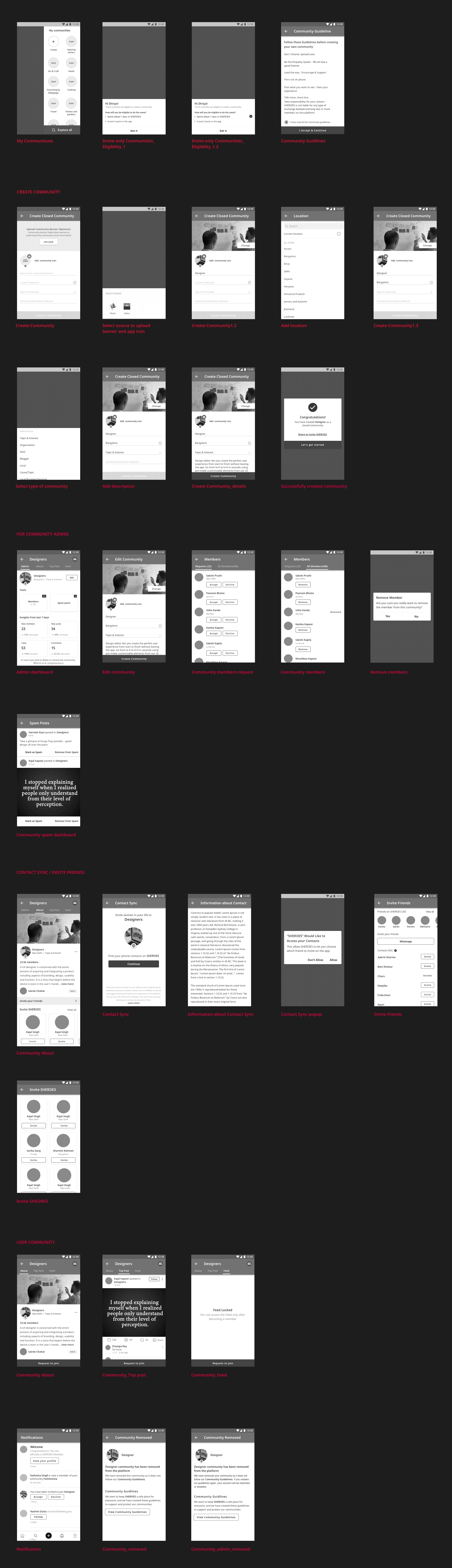The image showcases a series of overlapping pages against a solid black background, creating a somewhat organized yet chaotic visual. Most pages are in shades of white and gray, with some of the text displayed in white and visible, while other text remains obscured. 

Prominently, the top page displays the heading "My Communities," followed by "Invite Only Communities Eligibility 1.2" and "Community Guidelines," although the guidelines themselves are not visible in the image. Below, various prompts can be seen for creating and managing communities, including "Create Community," "Create Closed Community," "Select Source to Upload Banner and App Icon," and "Create Community 1.2." 

Further details include instructions to "Add Location," "Select Type of Community," "Add Description," and subsequently, a confirmation of having "Successfully Created Community."

The image also depicts different lists corresponding to community administrative tasks: 
- Admin Dashboard
- Add This Community
- Community Members Request
- Community Members
- Community Spam Dashboard

Additionally, there is a section for contact synchronization featuring:
- Invite Friends
- Information about Contact Sync
- Contact Sync Pop-Up
- Invite
- Pronouns: She or Hers

Another list pertains to regular user activities within the community, including:
- Community About
- Community to Post
- Community Feed
- Notifications of Community Removal
- Notification of Community Admin Removal

There is also a block of red text beneath the pages, the details of which are not specified in the description. The image captures the procedural aspects and layered intricacies involved in community management on a digital platform.